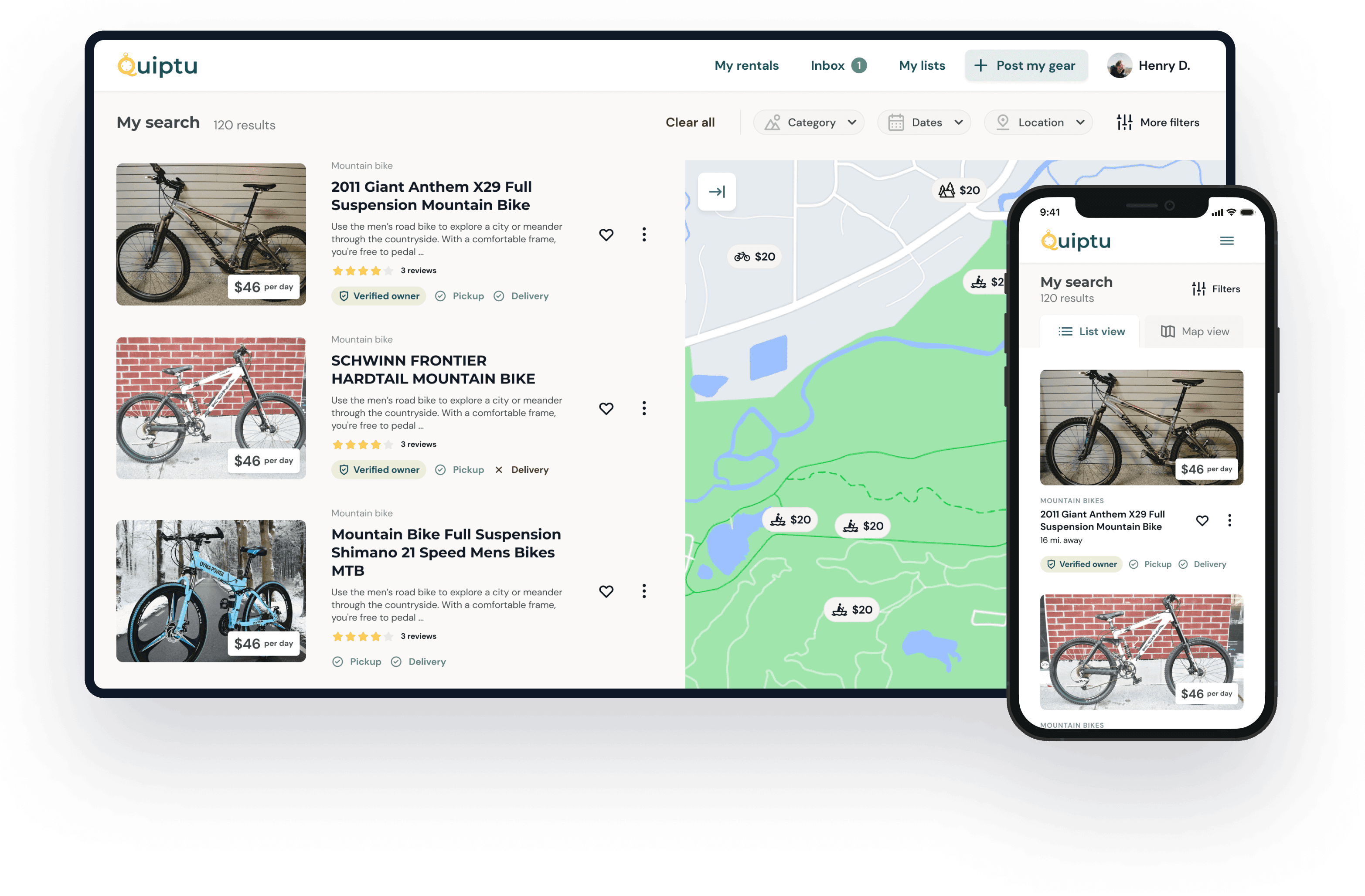This caption provides a detailed description of a screenshot showcasing both the website and mobile interface for Quip2, a platform dedicated to the rental of gear with a particular focus on mountain bikes.

**Caption:**
A detailed screenshot of the Quip2 platform is displayed, highlighting both web and mobile interfaces. The Quip2 logo is prominently positioned at the top left corner. Navigation links available include "My Rentals", "Inbox", "My List", and "Post My Gear." The logged-in user, "HenryD," is indicated at the top right accompanied by an icon.

The search results page shows the title "My search with 120 results," along with filtering options such as category, dates, location, and more. Each listing showcases an image of a mountain bike, a brief description, the price per day, and additional details like reviews, verified owner status, and options for pickup and delivery. Example listings include a 2011 Giant Anthem X29 full suspension mountain bike available for $46 per day, complete with three reviews, a verified owner status, and both pickup and delivery options. Another listing features a Schwinn Frontier hardtail mountain bike, also priced at $46 per day, with similar features and reviews. Additionally, there's a mountain bike with a full suspension and Shimano 21-speed men's bike, priced at $46 per day with three reviews.

On the right side of the interface, a map displays the locations of available mountain bikes, with price tags indicating their daily rental cost. The user interface appears intuitive and user-friendly, offering a straightforward list view or map view. Clear labels and icons enhance navigability, helping users make informed decisions efficiently.